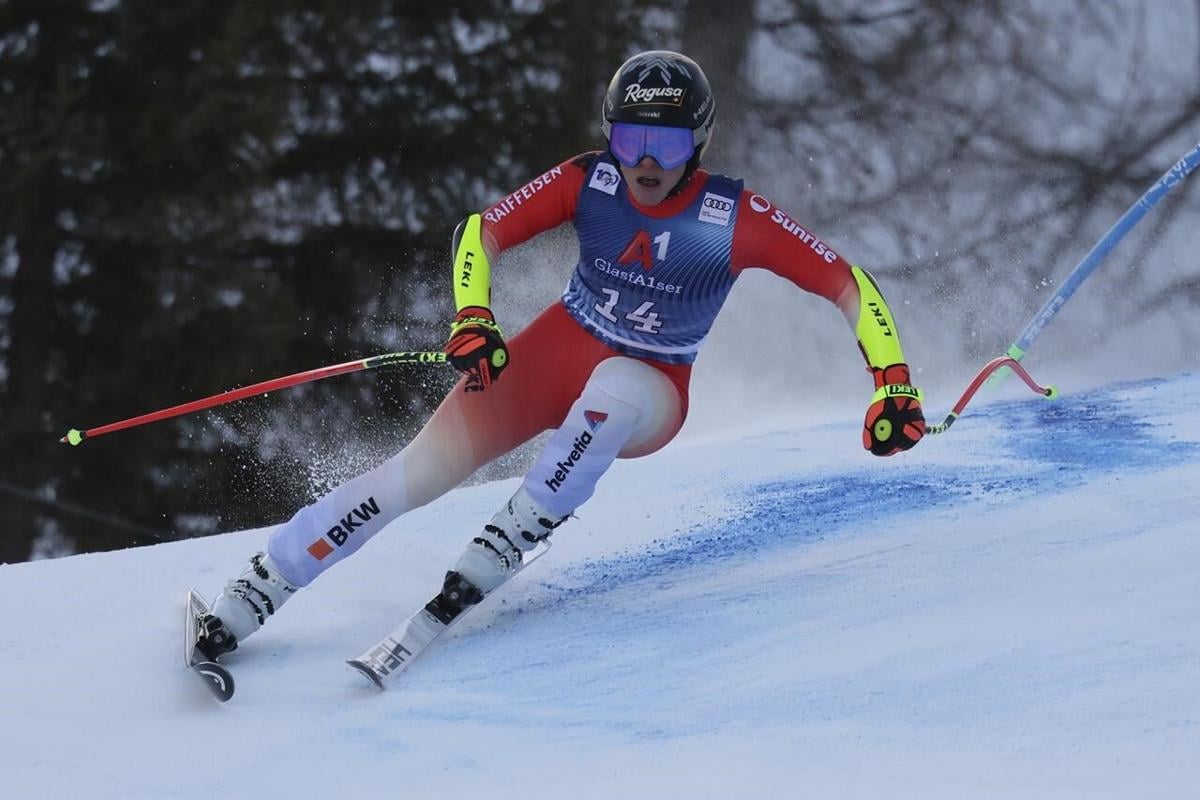The photograph captures a professional skier gliding down a slope in mid-action, with very minimal contact with the icy snow. The skier is dressed in a vibrant, colorful outfit that features fluorescent arms, red shoulders, and red leggings matched with a white and blue overall vest. The vest is adorned with various logos from sponsors such as Helvetica, BKW, Raiffeisen, and others. Skiing with red poles that have fluorescent tips and handles, the skier also sports purple goggles and a black helmet. While the gender of the skier is ambiguous, there is a suggestion that it might be a woman based on the physique. The skier's number, '14,' and possibly the name 'Glennisor,' is emblazoned on the outfit which also includes an Olympic symbol on one shoulder. The snow is densely packed and has a darker blue path marking the skier's trail, contrasting with the skier's colorful attire. The background features dark trees with sparse leaves, indicating a wintry, but not heavily snow-laden environment.